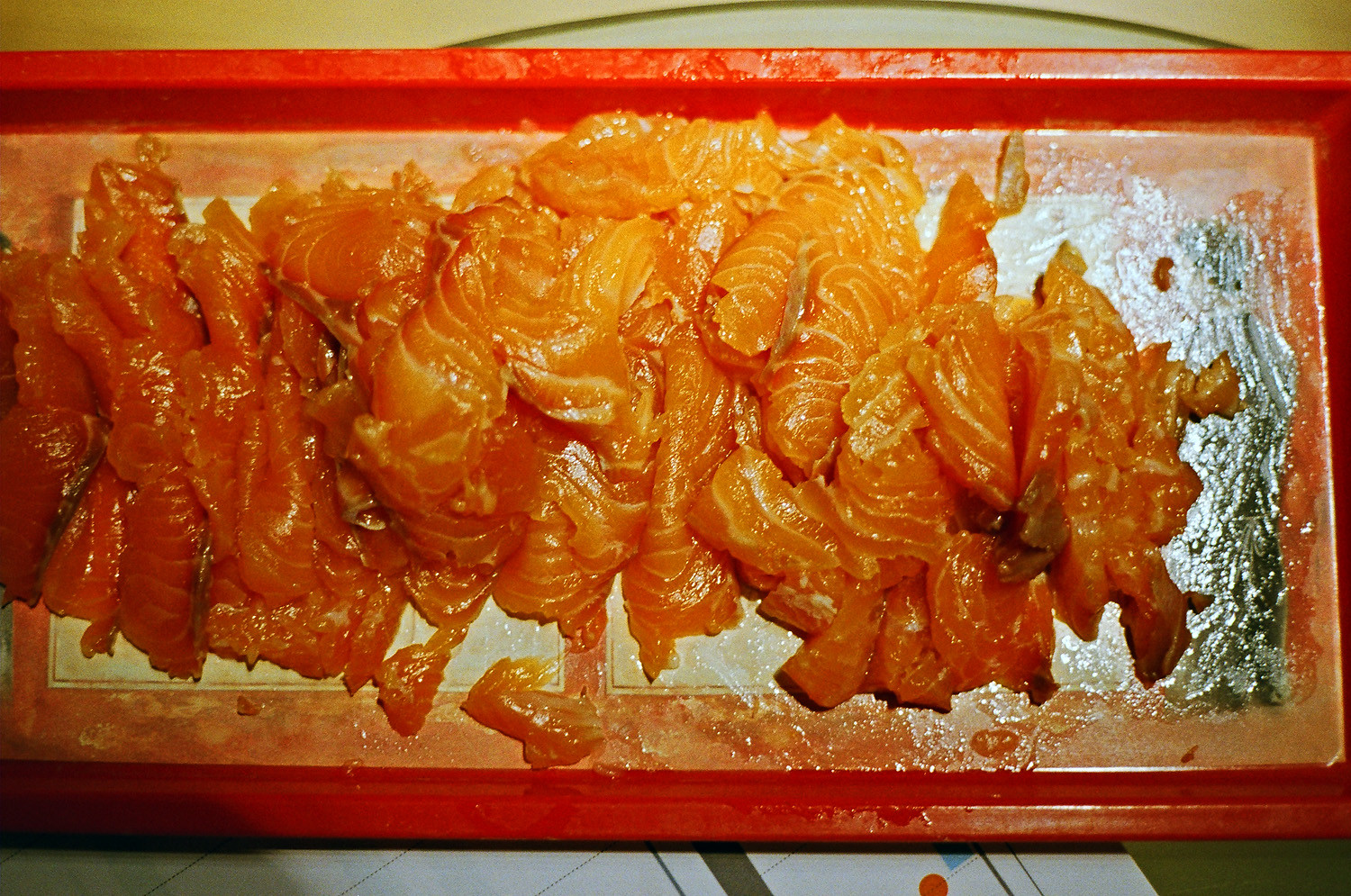The image displays a top-down view of a long, rectangular, orange tray, which is covered with an oblong pile of raw fish pieces. The fish appears to be a variety of types, as indicated by the differing shades of color — some pieces are a darker red while others are lighter with visible striations, suggesting muscle tendons. The meat is chopped and sliced into uneven, non-uniform pieces, and is very wet and oily, affecting even the top rim of the tray. The tray sits on a surface with a green and white background, possibly a counter, enhancing the overall vividness of the orange and red hues of the fish. There is also a small green image or object visible to the right of the tray.